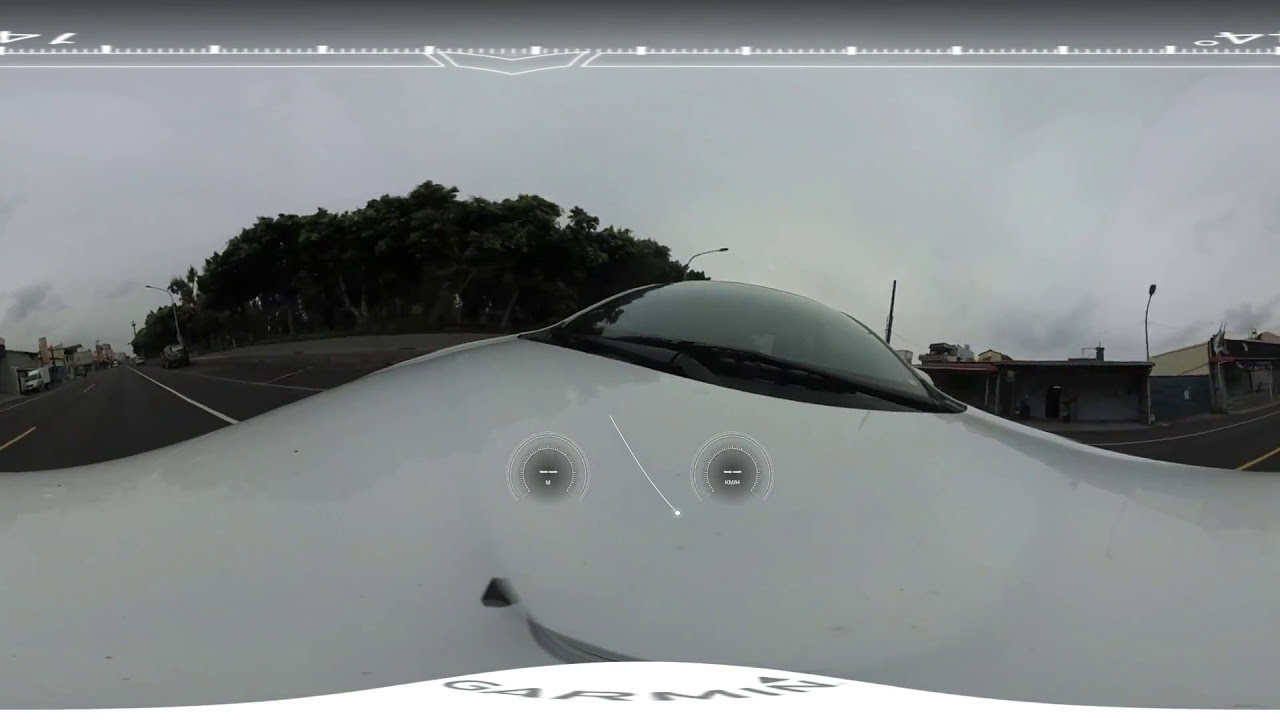In this intriguing photograph, we see what appears to be an altered image of a car designed to resemble a UFO on the road. Dominating the top of the horizontal rectangular image is a dark gray strip marked with white lines and numbers, giving the impression of an upside-down road. Below this strip, the actual road continues in dark gray asphalt, delineated with white dashed and solid lines, and flanked by mild traffic. A car with a sleek, metallic gray exterior, similar to a UFO, occupies the foreground. The car's hood features a playful design, with eye-like shapes and a smiley face. Above the hood, gray letters spell out “car men” on a white background. To the right side of the road, we see a cluster of green trees, a grassy area, and a collection of buildings housing various stores in tan, black, and red colors. Lampposts rise up amidst the scene, while the dreary, cloud-filled sky casts a gray hue over the entire image, adding to its edited, surreal atmosphere.